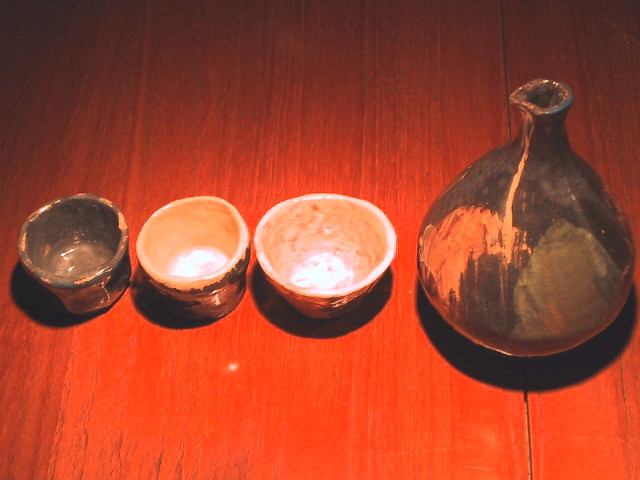In this photo, we see a collection of handmade pottery resting on an orange-toned wooden floor, which serves as the background. On the left-hand side, there are three small vessels: a blue bowl, a dark bowl with a white interior, and a slightly larger bowl that is predominantly white. All three seem to be made of clay and exhibit a shiny surface. The lighting casts large shadows beneath these objects, accentuating their shapes. On the right side of the image, there is a distinctive ceramic jug-like vessel. This jug features a spout at the top, suggesting it is designed for pouring. The surface of the jug is adorned with an array of colors including black, olive green, and a bright pinkish-orange, giving it a unique, albeit messy, appearance. There is no text in the photo, leaving the exact identity and purpose of these items open to interpretation.